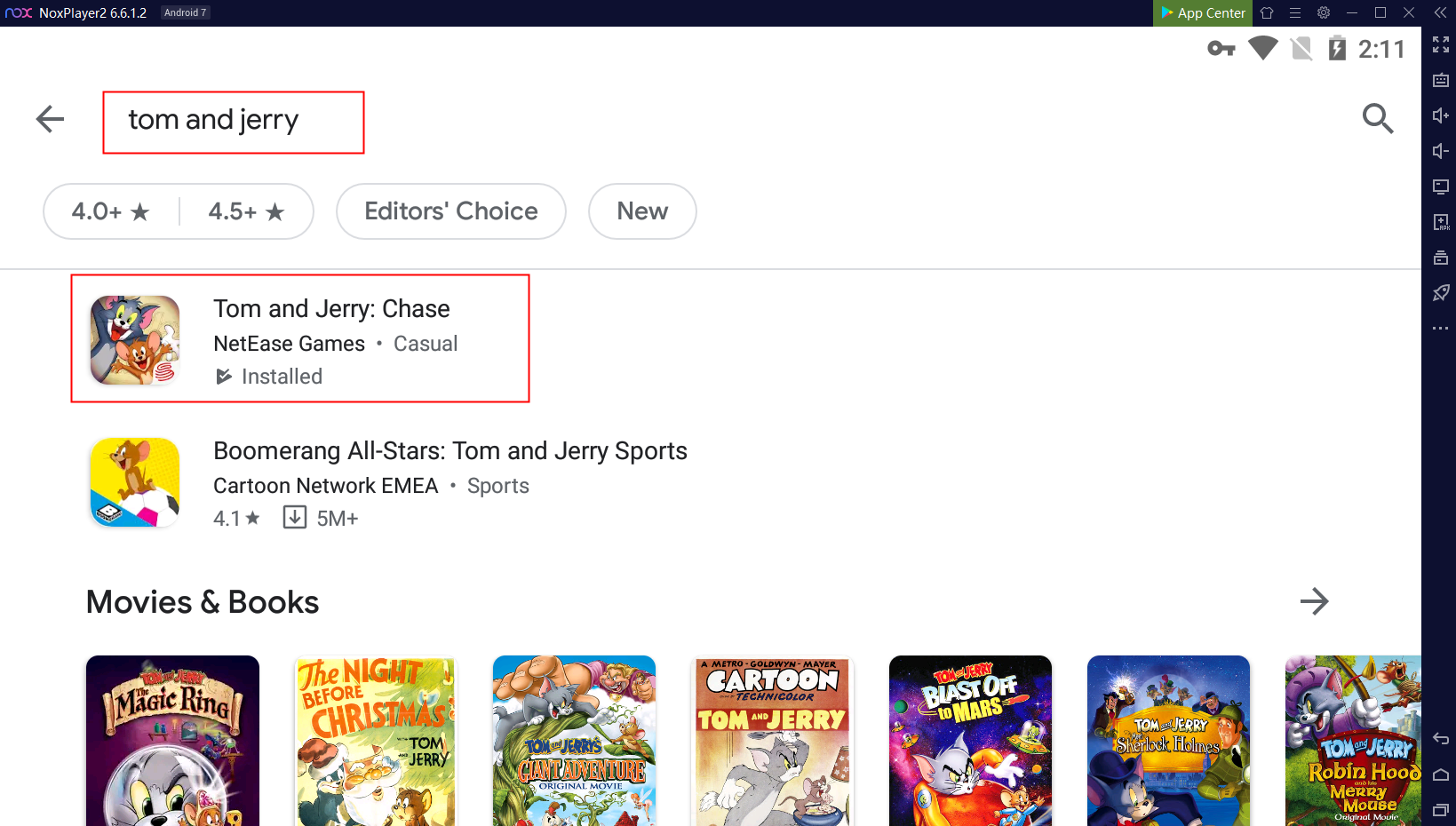In the image, we observe what appears to be an application page, presumably displayed on a tablet or smartphone, considering the presence of a status bar in the upper right corner showing the time (2:11), a battery charging icon, and Wi-Fi symbols. The overall design of the page is clean with a predominantly white background, black text, and several images. Certain sections are accentuated with red highlighting for emphasis.

At the top right, there's a navy blue pane featuring various icons. The first icon is highlighted in green and labeled "App Center." Adjacent to this, on the far left, a label reads "Next Player 2 6.612."

The main content of the page centers around a featured application, "Tom & Jerry Chase," surrounded by a red rectangle. Directly below this, the application is rated with "4.0 stars," "4.5 stars," "Editor's Choice," and marked as "New." Further details reveal the developer as "NetEase Games," the category as "Casual," and the status "Installed," also highlighted in red.

Below the featured section, there are recommendations for related apps such as "Boomerang" and "All-Stars" alongside "Tom & Jerry Sports," listed under the "Cartoon Network," and "EMA Sports," boasting a rating of "4.1 stars" and over "5 million downloads."

Towards the bottom of the page, a section titled "Movies & Books" showcases an array of visual thumbnails of various "Tom & Jerry" movies and books. The titles elucidated include "Magic Arena," "The Night Before Christmas," "Cartoon," "Tom & Jerry: Blast Off to Mars," and "Tom & Jerry: Robin Hood."